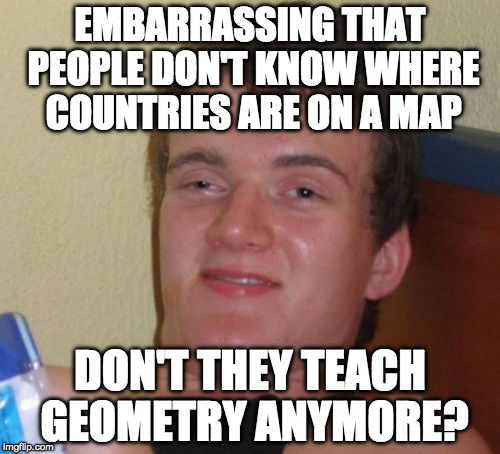A middle-aged white male with light skin and partially closed eyelids, giving a relaxed expression, is the focal point of this image. He is looking slightly off to the left rather than directly at the camera. The background features a very light brown or cream-colored wall to the left of his face and what appears to be a headboard made of wood, partially painted blue, to the right. Additionally, there is a clear plastic bottle with a dark blue cap and a light blue stripe along its side, positioned on the left edge of the image. Text overlaying the image reads, "Embarrassing that people don't know where countries are on a map. Don't they teach geometry anymore?" in bold white letters with a black outline. The surrounding environment suggests an indoor setting, potentially with a style indicating a bedroom, evidenced by the possible headboard and the bottle. The man's appearance includes brown hair, and the photograph captures him from the shoulders up. The image credits "imgflip.com" are visible beneath the bottle.